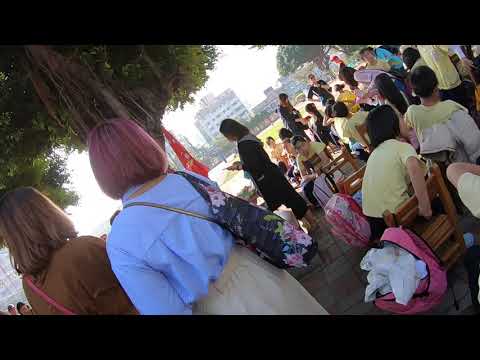The image captures a lively outdoor gathering, possibly in a park or an urban setting, taken at a diagonal angle. The foreground features the backs of two females standing near a large tree, one with light brown hair and wearing a brown shirt, while the other has short reddish hair and dons a light blue blouse with beige bottoms, holding a floral print bag on her right shoulder. To their right stands another woman in a black dress, observing something in her hands. Further to the right, rows of collapsible wooden chairs are lined up, some occupied by children in yellow t-shirts who are busily moving around. In the lower right-hand corner of the image, an open pink backpack reveals some white bags. The scene is bathed in bright daylight, with silhouettes of buildings visible in the distant background, suggesting an urban environment. A red flag or similar item hangs near the tree, adding a touch of color to this vibrant assembly.